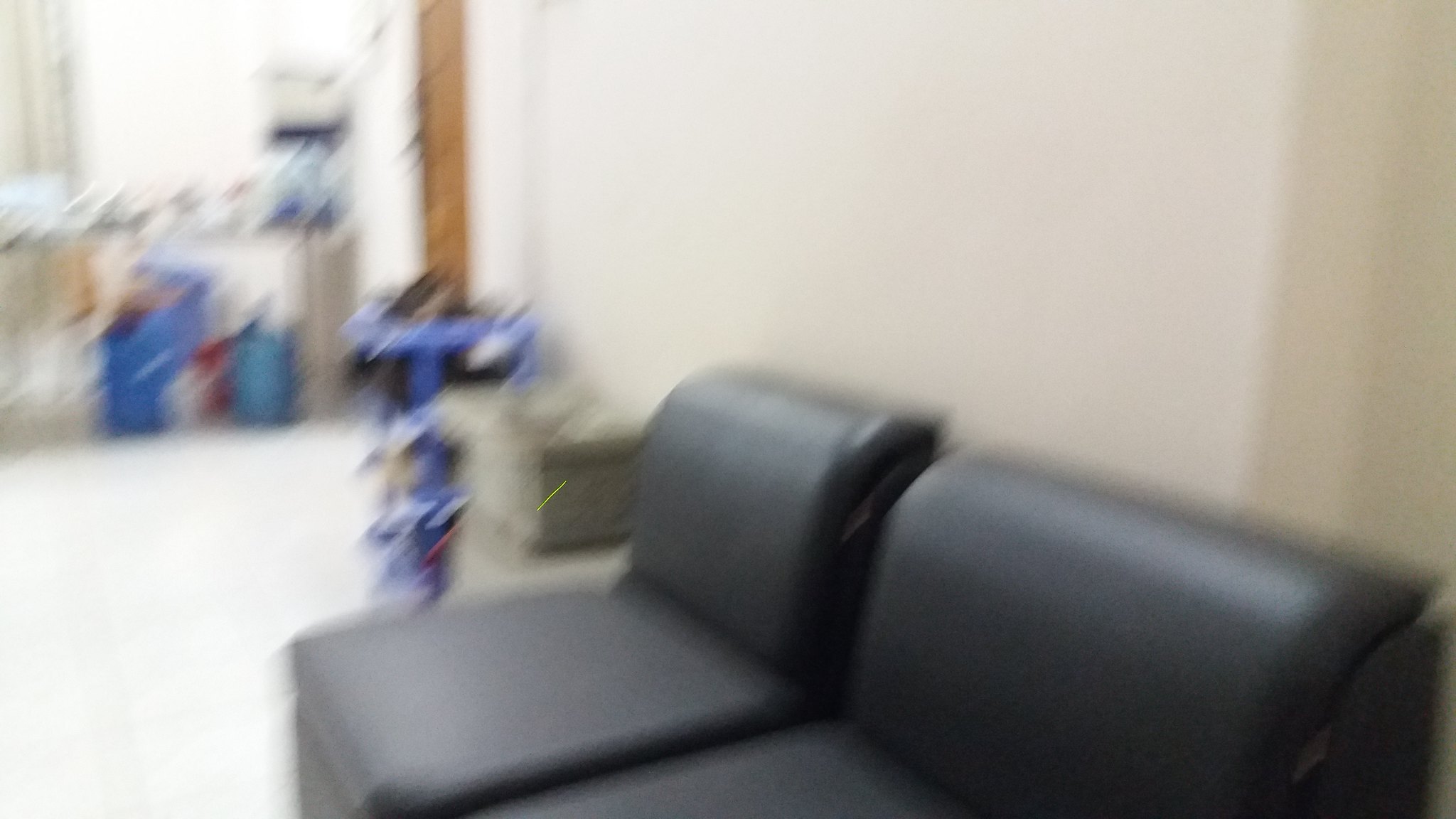This image captures a very blurry photograph of an indoor room dominated by a modern black leather sectional couch with noticeable curvature at the back and no armrests. The couch consists of two seats with smooth black leather and rectangular seat cushions. Behind the couch, there's a white wall and a white floor which appears to be tiled. To the right of the seating, some indistinct, blurry objects can be seen, including a blue vertical rectangle and a perpendicular shape that might be part of shelving or a piece of furniture. A brown wooden plank can also be identified in the background. There is a combination of some blue, white, off-white, and red items, possibly boxes, adding a contrasting splash of color to the otherwise monochromatic room. Additionally, a window on the back left side of the room emits a bright white light, further obscuring the details of objects placed in front of it.